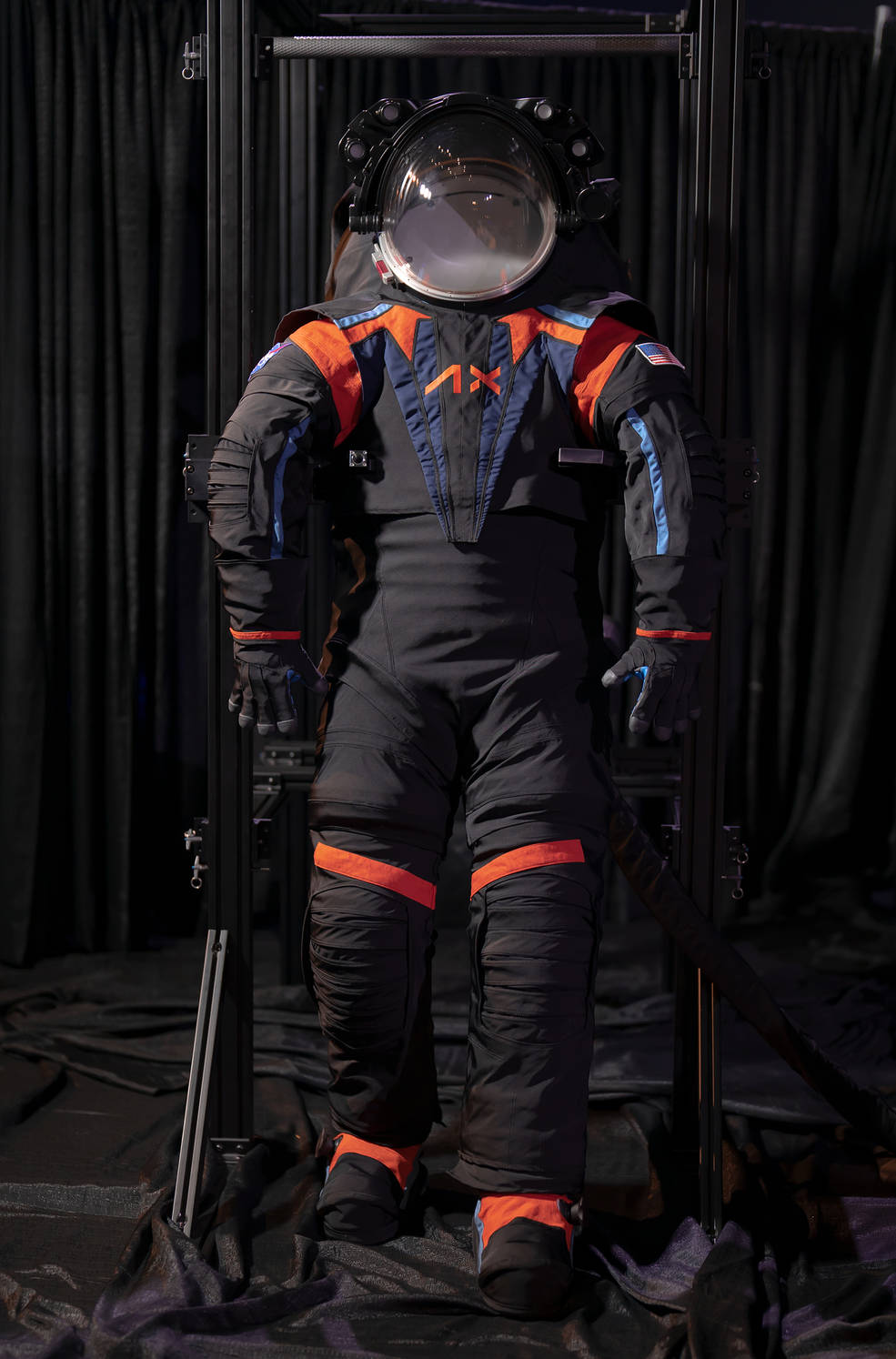The image showcases a futuristic astronaut suit, meticulously arranged as if an astronaut is wearing it, though it is unoccupied. The suit boasts a predominantly black color scheme, accented with striking orange and varying shades of blue details concentrated on the knees, ankles, upper chest, and wrists. A clear glass shield fronts the helmet, complemented by a large black apparatus encircling the upper head. The suit includes black braces, possibly for securing the astronaut in space. It is displayed against a backdrop of a dark curtain, with shiny black fabric covering the ground beneath, creating an elegant setting. Additional elements like gloves and shoes are part of the ensemble, with a pack on the back resembling an oxygen system. The suit is propped up with support apparati, including a square cage-like structure, and is highlighted by strategic lighting that emphasizes its modern, high-tech appearance.